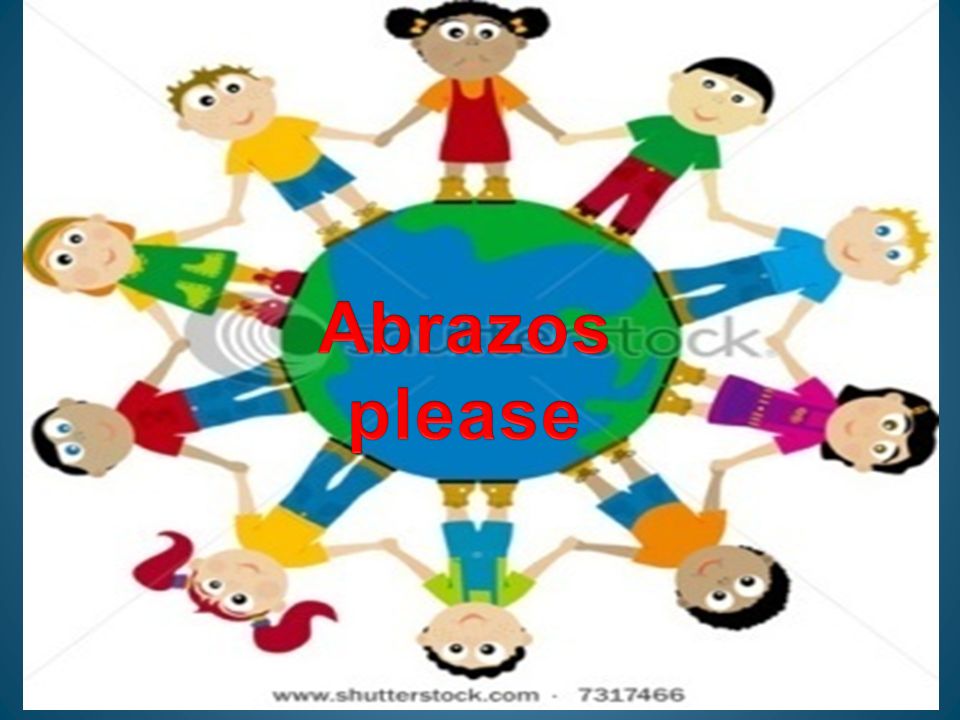The image depicts a colorful, cartoonish illustration with a white background. Central to the image is a simple drawing of the Earth, represented with blue and green. Surrounding the globe are ten diverse cartoon children holding hands, forming a circle around the Earth. These children vary in complexion and ethnicity, each wearing different colorful outfits – including a girl with an orange shirt and red dress, a boy with a green shirt and purple pants, a blonde boy in a blue shirt and jeans, and another girl with red hair. Each child stands on the Earth, with the children at the bottom appearing upside down to maintain their hold in the circle.

In the center of the Earth, red digital text reads "ABRAZOS, PLEASE." At the bottom of the image, there is a watermark text "www.shutterstock.com" along with the identification number "7317466." Additionally, there is another Shutterstock watermark in the middle of the image, without the ".com" suffix. The overall style is vibrant and playful, emphasizing unity and diversity among children.